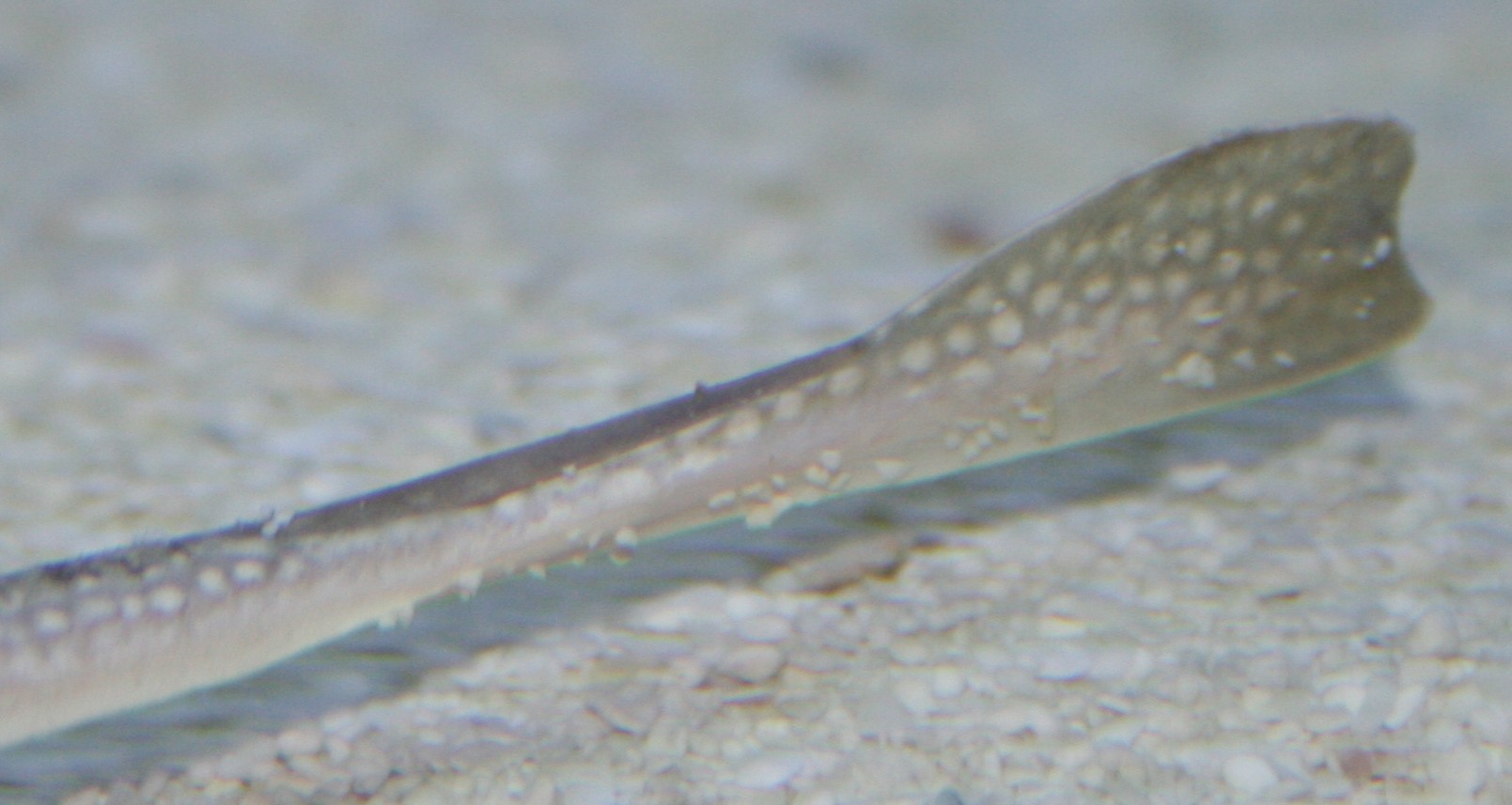In this underwater scene, the focal point is a light gray, narrow, scaly tail with faint white spots, likely belonging to a fish or possibly a stingray, given its subtle fin at the end. This tail, which darkens slightly to a brownish hue towards its tip, swims through a backdrop of fine-grained sand and small pebbles, indicating its aquatic environment. The background is a bit blurry but the immediate foreground, where the tail is, remains clear, highlighting the intricate details of its scaly surface and the pattern of spots.